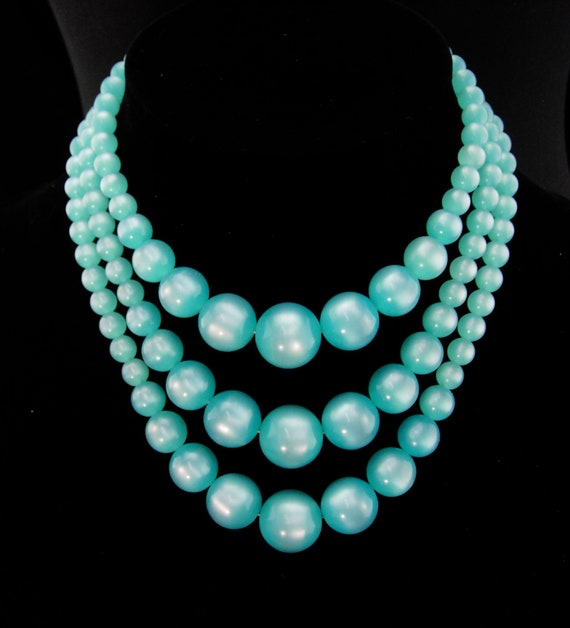The photograph showcases an elegant necklace composed of three strands of pearls, delicately draped around a dark mannequin neck, which serves as the background. Each strand contains approximately 30 light aquamarine, jade-colored beads that gradually decrease in size from the larger central beads to the smaller ones near the clasp. The pearls exude a notable shine, with a white sheen more pronounced in the upper left corner of the image, enhancing their lustrous appearance against the stark black backdrop. The overall presentation highlights the intricate craftsmanship and the stunning visual contrast between the vibrant pearls and the dark display.